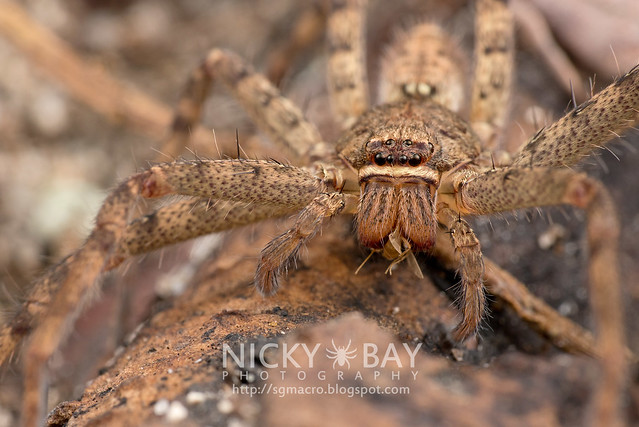The image is a professionally taken, full-color, extreme close-up photograph of a large spider, possibly a tarantula. Captured outdoors using natural light, the square image is devoid of borders and features a predominantly brown, out-of-focus background. The spider, poised on what seems to be a log, commands the viewer's attention with its intricate details: eight glossy black eyes arranged in rows, prominent fangs possibly holding a smaller insect, and bristly hair covering its body and eight legs. The spider itself is a light tan with dark brown spots and some black markings down its legs. At the bottom center of the photograph, there's a watermark in white text that reads "Nicky Bay Photography" flanked by a small drawing of a spider, followed by the website "http://sgmacro.blogspot.com."